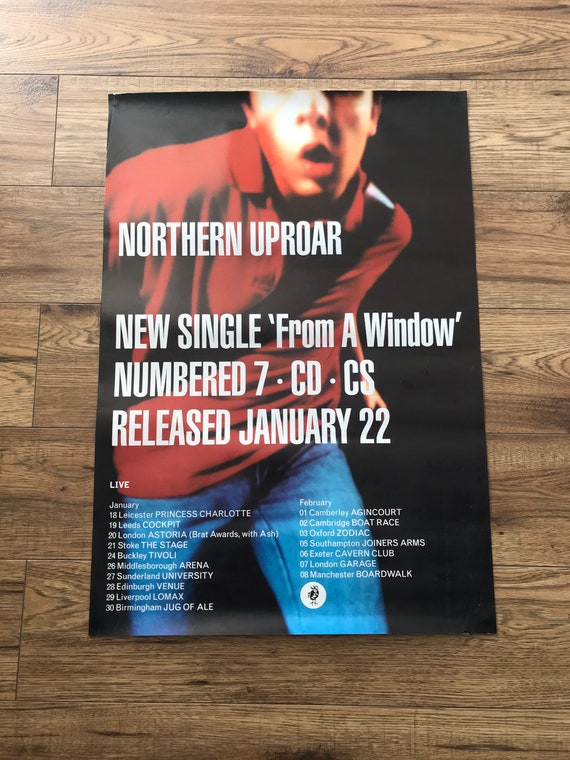The image depicts a vertically oriented, realistic-looking photograph set against a background of wooden boards, which could either be a wall or a floor made of light wood planks. In the center, there is a rectangular, vertically oriented poster with a black background. The poster features a close-up shot of a young white man, possibly in his late teens to early 30s, wearing blue jeans and a red collared shirt. Only his face from the chin to the eyes is visible, giving the impression that he is moving towards the viewer. This man also has a strap across his chest, suggesting he might be carrying a guitar or a bag.

In white text on the poster, it says, "Northern Uproar, our new single, 'From a Window', numbered 7, CD and CS, released January 22nd." Below this, there are additional lines that likely list concert dates, with mentions of both January and February. The detailed layout and minimalist design emphasize the promotional nature of this music poster.